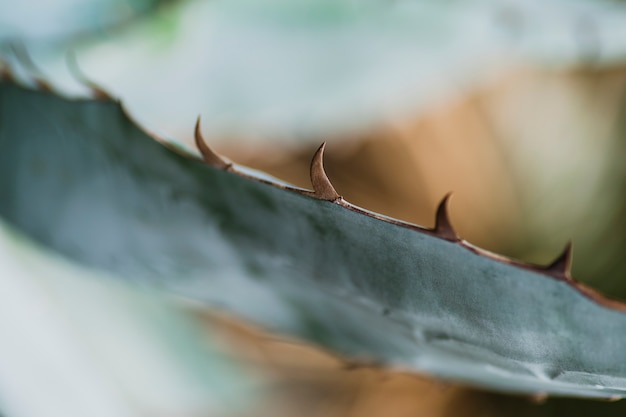The image features an extreme close-up of a single gray-green leaf with a distinctive texture. Notably, the rightmost edge of the leaf is adorned with sharp, brown thorns that resemble rosebush thorns or curved canine teeth, displaying a gradient from light brown to dark brown depending on the lighting. The leaf itself has a hint of aquamarine and transitions from white at the front to almost black at the bottom right corner. The leaf stretches diagonally from the upper left to the lower right of the image. The background remains unidentifiable due to its blur, containing indistinct patches of white, green, brown, and beige. This blurriness amplifies the leaf’s detailed and textured edge, emphasizing the thorny pattern along its side.